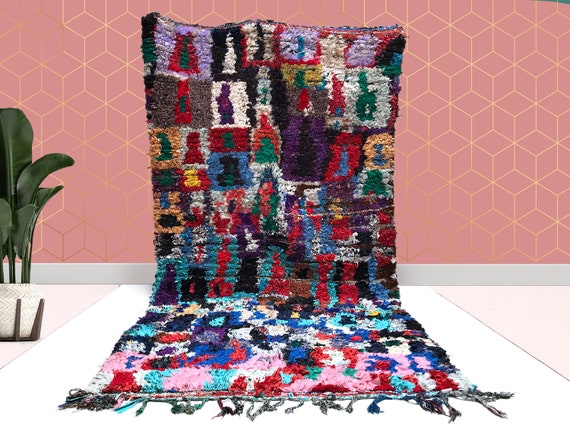The photograph captures a highly artistic DIY rag quilt, prominently displayed against a pink wall adorned with golden cubic patterns. The quilt itself, a vibrant patchwork of colors—white, red, pink, blue, yellow, brown, and black—stretches vertically up the wall before cascading down to the floor and moving towards the camera. The intricate stitching and varied hues create an abstract, splotched mosaic, with rectangular shapes and representations of figures and objects embedded within. The quilt features a rough, jagged fringe along its base, adding a rugged texture. The room's white baseboard and light gray floor are visible at the bottom, while a bright green, large-leafed plant sits to the left in a white vase with jagged patterns, supported by a brown wooden stand. This dynamic composition contrasts the quilt's chaotic beauty with the geometric precision of the room's decor.